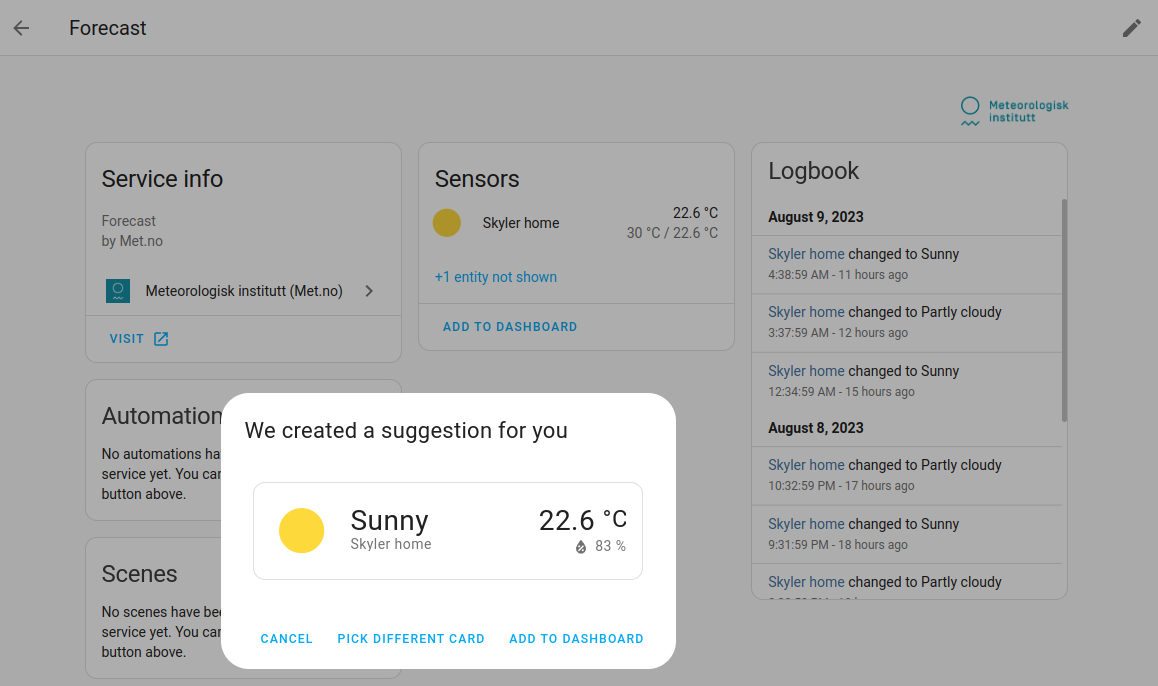This is a left-to-right horizontal image featuring a user interface with a grayed-out background. The background is slightly muted to highlight a white pop-up box at the center. Despite the white box's prominence, the rest of the interface is discernible, except for areas obscured by the pop-up.

**Background Details:**
- In the upper left-hand corner, there is a backward-pointing arrow, likely a navigation or back button.
- On the right-hand side, an icon is displayed, beneath which lies the label "Meteorologist Institute" in a bluish-green hue accompanied by a small icon.
- Various option boxes are present, labeled "Service Info," "Sensors," "Logbook," "Automation," and "Scenes." However, the bottom parts of the "Automation" and "Scenes" boxes are partially hidden by the pop-up box.

**Pop-up Box Details:**
- The white pop-up box is rectangular with rounded edges and occupies the center stage of the interface.
- Within the pop-up, black text states, "We created a suggestion for you."
- Another rounded, long horizontal box is nested inside the white pop-up. It contains a yellow circle and the text "Sunny, Skyler Home, 22.6 degrees Celsius." 
- This nested box also indicates a probability, showing "83%," likely for the chance of rain.
- At the bottom of the pop-up, there are three blue options: "Cancel," "Pick a different card," and "Add to dashboard."

Overall, the image showcases a weather-related user interface screen, where the central focus is on a pop-up suggesting a weather update, enhancing user interaction with options to manage the displayed information.